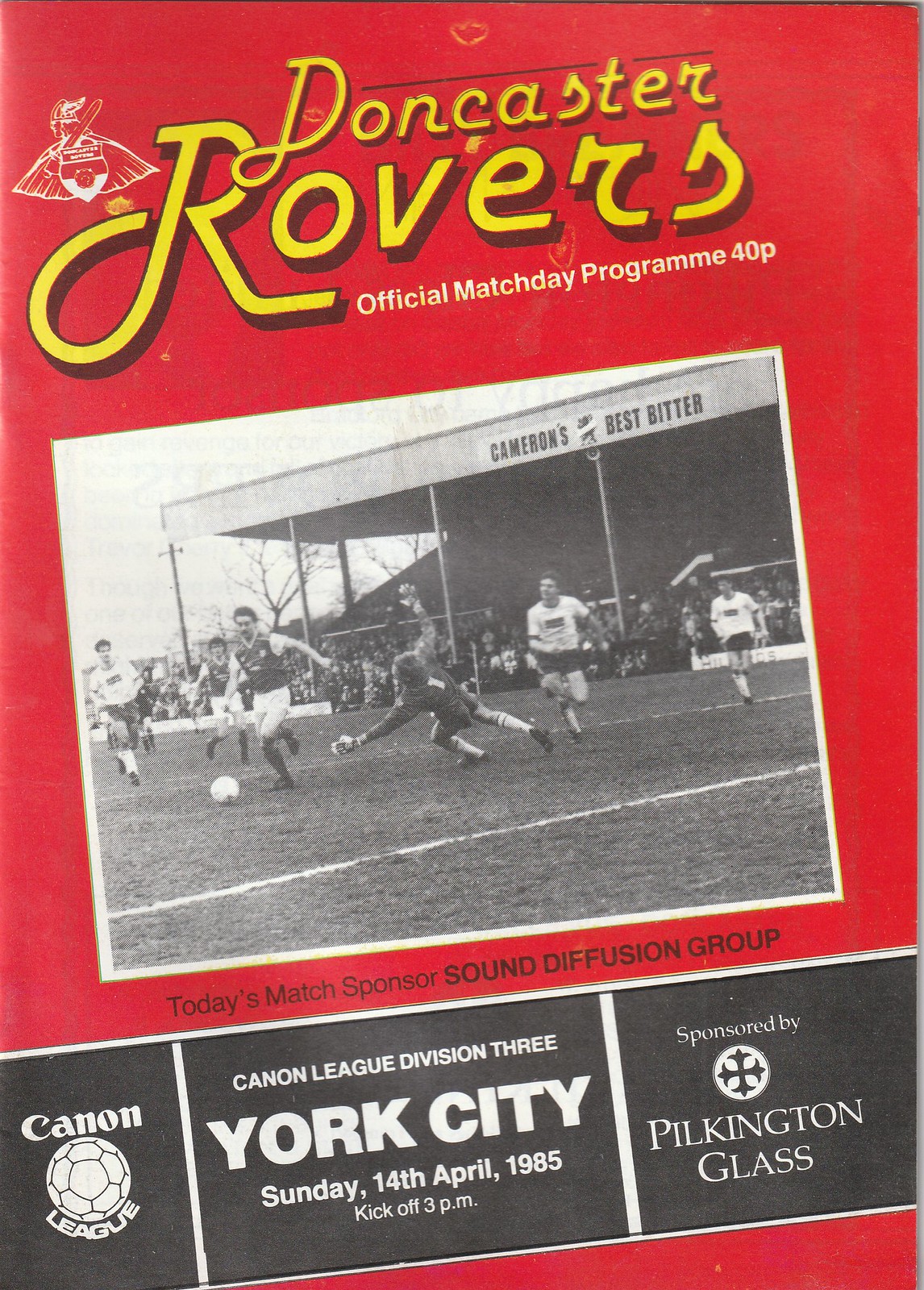The image is a color scan of a soccer program cover, with a vibrant red background. Dominating the top in a yellow, vintage-style font, the text reads "Doncaster Rovers," with "Doncaster" in smaller letters and "Rovers" in a larger, bold script. Directly below, in small white text, it states, "Official Match Day Program 40P." The program features a diagonally tilted black-and-white photograph of a soccer game, positioned lower on the left and higher on the right. The image captures a dynamic moment where a goaltender is diving to stop the ball, with several other players in the background. Below the photo, in bold black text, it reads, "Today's Match Sponsor, Sound Diffusion Group."

At the bottom of the cover, a three-sectioned black stripe runs horizontally. The left section features the Cannon League logo beside the words, "Cannon League." The middle section details the event: "Cannon League Division III, York City, Sunday, 14th April, 1985, kickoff, 3 p.m." The right section mentions another sponsor: "Sponsored by Pilkington Glass," accompanied by the company's logo. The program also includes an emblem in the upper left, depicting a man with a sword, broad wings, and a shield.